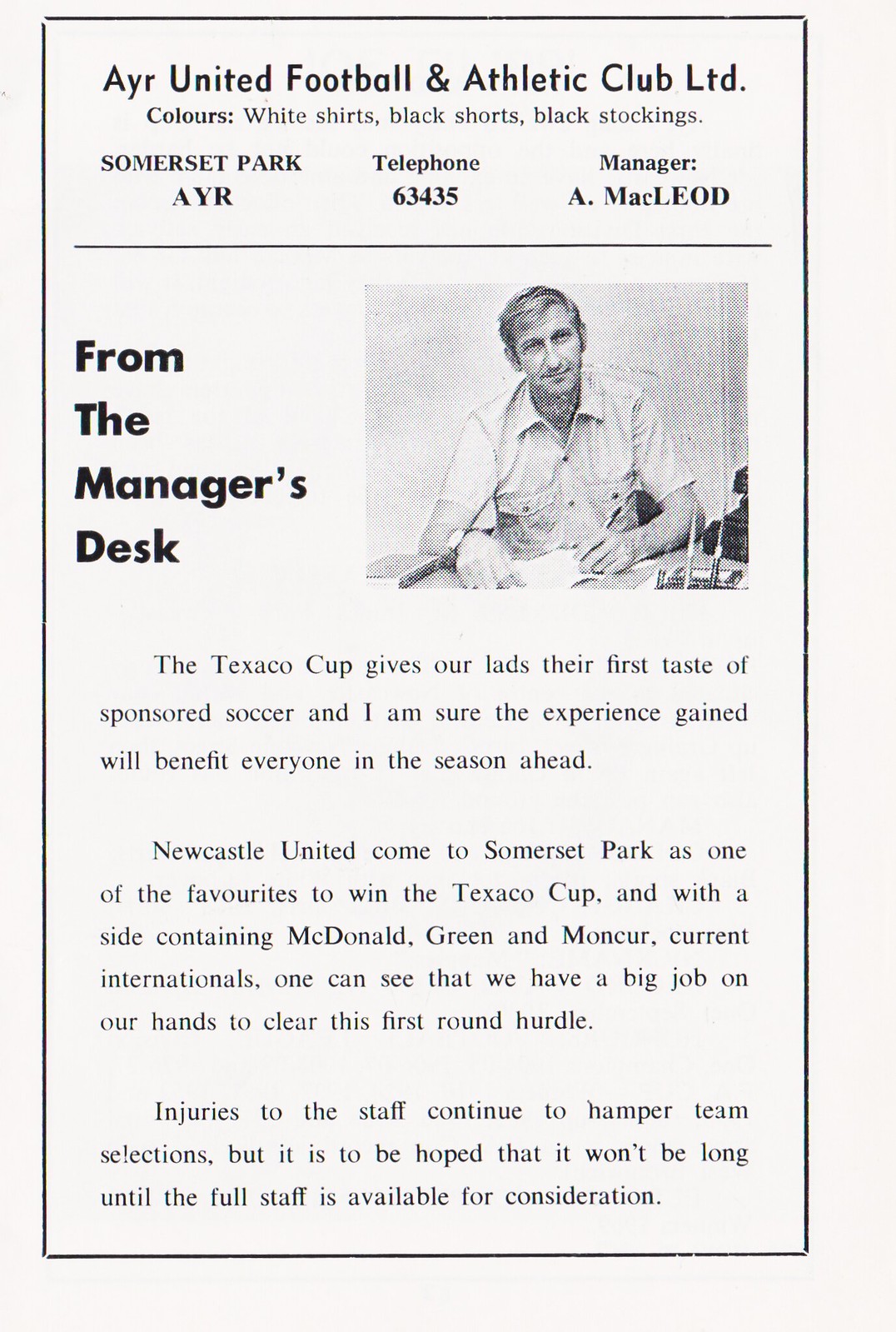This image appears to be a vintage black-and-white newspaper clipping or flyer from AYR United Football and Athletic Club Limited. It prominently features the club's details: "Colors: White Shirts, Black Shorts, Black Stockings," "Somerset Park, AYR," and "Telephone 63435." The manager is listed as A. MacLeod. On the right-hand side, there's a photograph of a man in a collared button-down shirt, holding a pen in his left hand and writing in a notebook while sitting at a desk. The desk has a pen stand and a book, and the man is looking straight at the photographer. The headline reads, "From the Manager's Desk." Below, there's an excerpt stating: "The Texaco Cup gives our lads their first taste of sponsored soccer, and I'm sure the experience gained will benefit everyone in the season ahead. Newcastle United come to Somerset Park as one of the favorites to win the Texaco Cup, and with a side containing McDonald, Green, and Munro, current internationals, one can see that we have a big job on our hands to clear this first round hurdle. Injuries to the staff continue to hamper team selections, but it is hoped that it won't be long until the full staff is available for consideration."